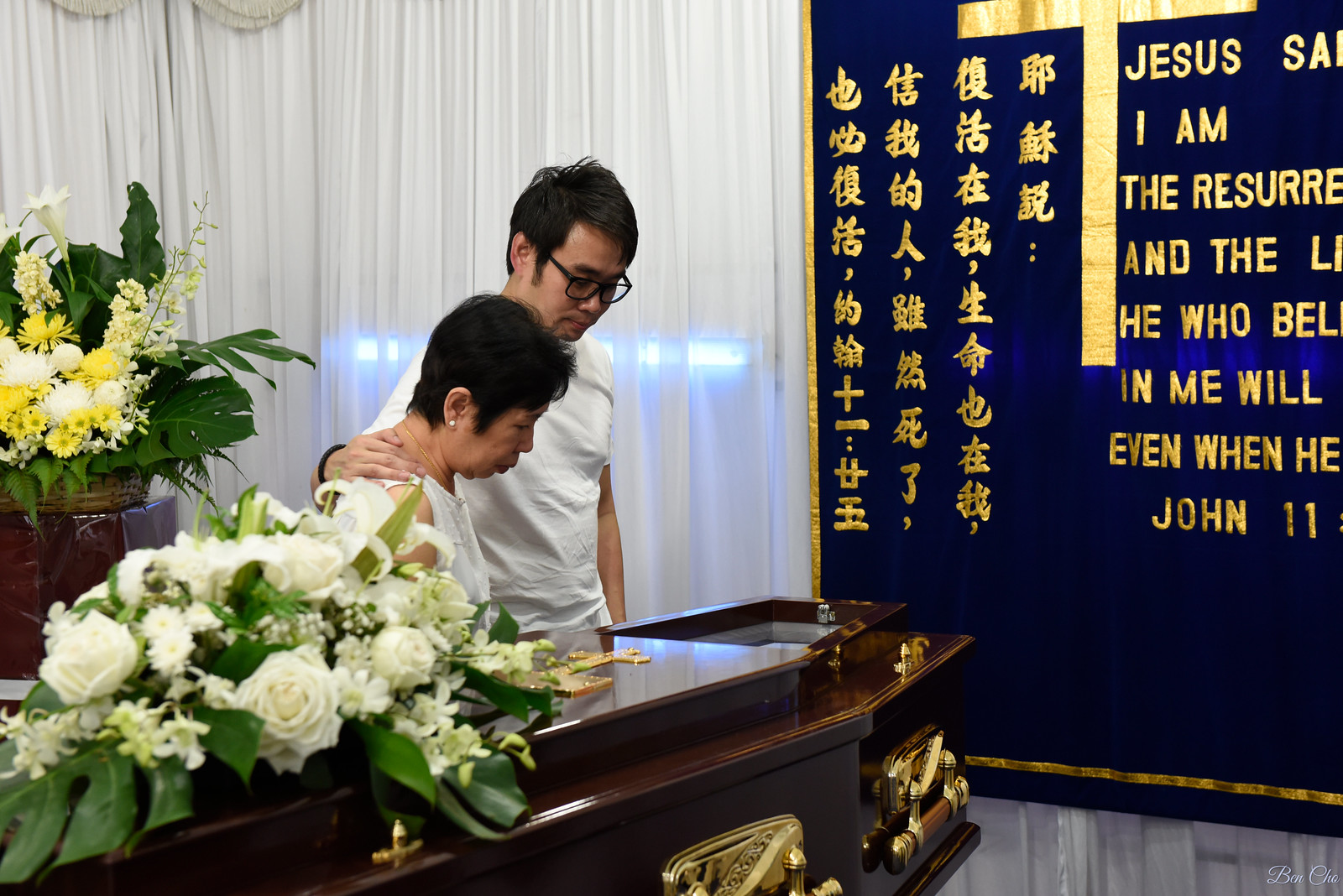This photograph captures the solemn scene of an indoor funeral, likely in an Asian country. Dominating the frame are an older Asian woman and a younger Asian man, both dressed in white—an indication of mourning. They stand in front of a dark wood casket adorned with gold fixtures and topped with a large bouquet of white roses. Behind this primary scene, another bouquet composed of yellow and white flowers with large green leaves is visible. A distinctive blue tapestry with gold Chinese lettering and biblical text, including the partial quote "Jesus said, I am the resurrection and the life," and reference to John 11, hangs in the background. White curtains frame the window, adding to the somber yet sacred atmosphere.